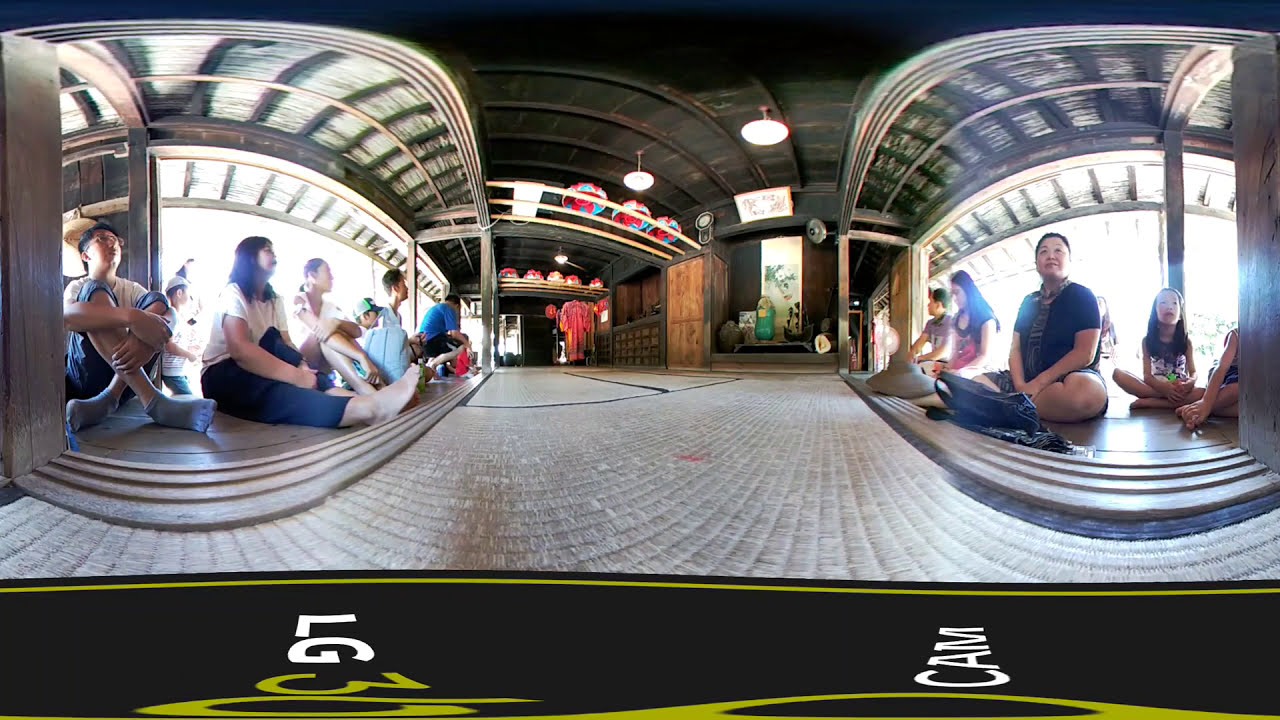The photograph depicts the interior of an old, possibly Asian temple, captured with a 360-degree fisheye lens, creating a distorted view that curves inward toward the center. The floor appears to be either tiled or made from a wood-like material, while the ceiling is made of brown wood or bamboo, adorned with umbrella-shaped light fixtures. A text in white and yellow at the bottom of the image reads "LG 360 cam" against a black background.

The scene shows various people sitting on the ground along the edges of the room, facing each other and towards the camera. Many of them have removed their shoes, with some barefoot and others wearing socks. The group appears to be of different ages, and most of the individuals seem to be Asian. The central area of the temple is empty, potentially reserved for religious or ceremonial purposes, with some religious figures or stands visible in the background. The overall ambience suggests a serene, observant setting, with the people likely engaged in a form of ritual or ceremony.